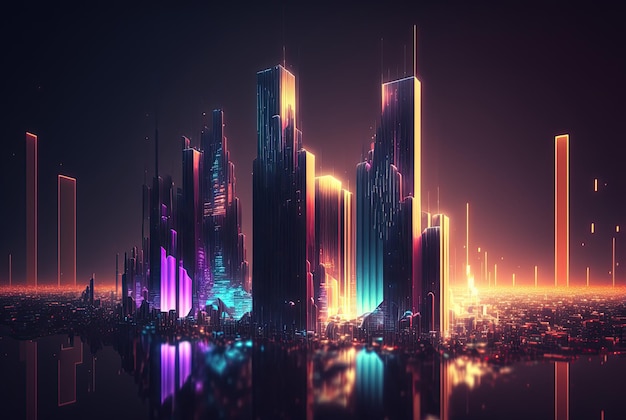This is a digitally created image of a futuristic cityscape at night. Dominating the scene are numerous tall skyscrapers, predominantly seen in purple and blue hues. The tallest skyscrapers are in the center, while smaller buildings are positioned toward the edges of the composition. 

The city's vivid neon lights reflect off what appears to be a body of water at the bottom of the image, enhancing the vibrant colors. On the left side, buildings are bathed in purple, transitioning to blue structures, and then to a striking black building with blue vertical stripes. As your eyes move further right, a more diverse array of structures comes into view, painted in yellowish, blue, and black tones, highlighted by their vibrant, fluorescent lights.

On the far right, there's a large, rectangular portal-like structure in a bold red with a yellowish background, contrasting sharply with the rest of the cityscape. Similarly, a sizable dark brown portal-like shape with pink borders stands on the left, adding to the visually arresting, almost science-fictional aesthetic of the scene. The backdrop is enveloped in darkness, punctuated by city lights, silhouettes, and subtle hues of purple and yellow, creating a captivating, futuristic atmosphere.